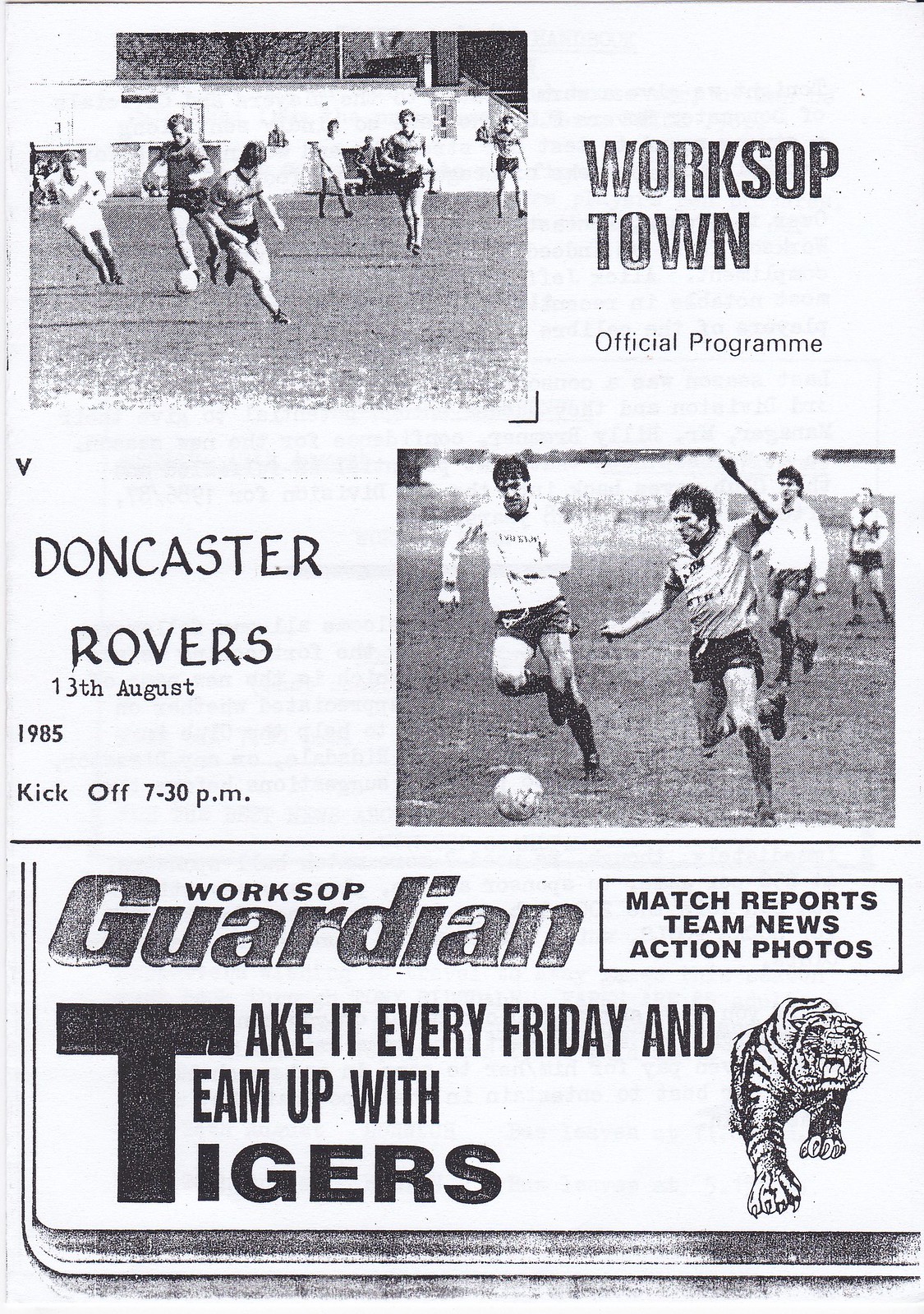The image is a full-page, light blue advertisement for a soccer game featuring Doncaster Rovers. The top third of the page showcases a black-and-white photograph of multiple soccer players in action on a field with a building visible in the distance, filtered with a blue tint. To the right of the photo, large uppercase text reads "Workshop Town," followed by "Official Program" in smaller print. The middle third features another black-and-white photo of four players preparing to kick a soccer ball, positioned on the right side. On the left, large print states, "Doncaster Rovers," and beneath it, in smaller text, "13th August 1985, kickoff 7.30 PM." The bottom third of the page has a prominent headline, "Workshop Guardian," and an invitation in uppercase letters to "take it every Friday and team up with Tigers." A drawing of a tiger with claws extended is situated on the right, next to a text block listing, "Match Reports, Team News, Action Photos." The advertisement appears to be a scanned version of an original promotional pamphlet.